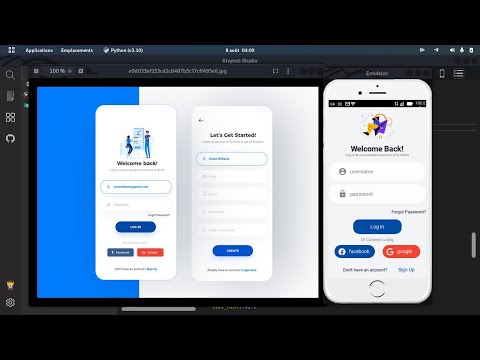A meticulously designed web page features a black background, with the main content area centered and set against a dark gray backdrop. Dominating this section is a large square window. Adjacent to this window on the right is the image of a cell phone, which is split into a blue background covering one-third of the area and a white background occupying the remaining two-thirds. This image includes two rectangular pop-ups: the top one contains a text input bar with a blue login button below it, followed by a blue Facebook tab and a red square to its right. 

To the right of this setup, there is another image depicting a rectangular screen displaying the text "Let's get started," a prominent search bar beneath it, and a blue button at the bottom. 

Further right is an image of a white phone screen featuring a welcome message at the top. This screen prompts users to input their username and password, followed by options to log in via a traditional login button, a Facebook button, or a Google button.